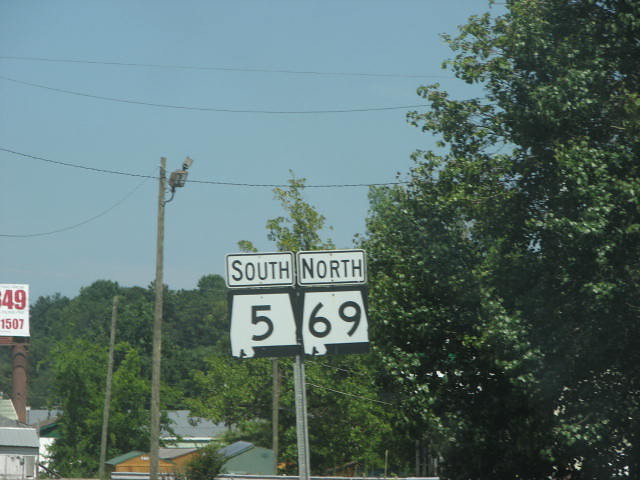Under a pristine blue sky crisscrossed by utility wires, an image captures a snapshot of a neighborhood at the intersection of Texas Highways 49 and 1507. To the left, an electrical pole stands tall adjacent to a white sign. In the background, residential buildings with grayish-blue rooftops and brown walls create a picturesque suburban scene. The right side of the image is dominated by lush green foliage, showcasing the vibrant leaves of multiple trees. 

At the very center, a metal pole holds up a rectangular white sign with black text, indicating directions: "South" on the top left, "North" to the right of it, "5" below on the left, and "69" on the right. Toward the bottom left of the image, there is a person engaged in an activity that resembles mining or digging into a hillside, making a noticeable cutout into the terrain.